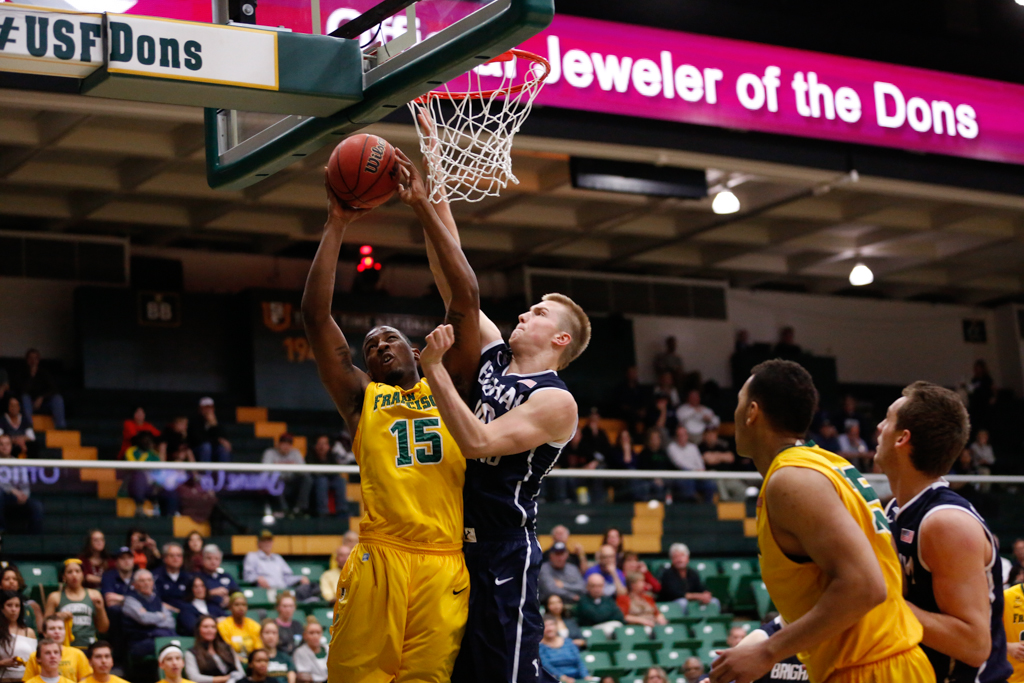The image captures an intense moment in a basketball game, with vivid details of the action and the setting. In the center, an African American player wearing a yellow uniform with the number 15 is leaping towards the basket, holding the basketball with both hands as he attempts to score. His determined posture suggests he's about to dunk the ball. Directly opposing him, a Caucasian player in a dark blue uniform is also airborne, his right hand extended in a defensive attempt to block the shot. Below and around the main players, two more athletes are engaged in the action - one teammate of the player in yellow and one teammate of the player in blue, both standing about four feet away and watching closely. 

The background showcases the arena setting with stands partially filled with spectators, some sections revealing empty green and blue seats, indicating a moderately attended game. Above the crowd, a purple banner prominently displays the words "Official Jeweler of the Dons" in white text. Additional glimpses of advertisements such as "OfficeMax" and logos linked to "USF Dons," likely indicating the University of San Francisco team, add to the professional atmosphere of this basketball game. The slightly blurred audience fixes their gaze on the riveting play unfolding before them, amplifying the drama of the moment captured just before the scoring attempt.